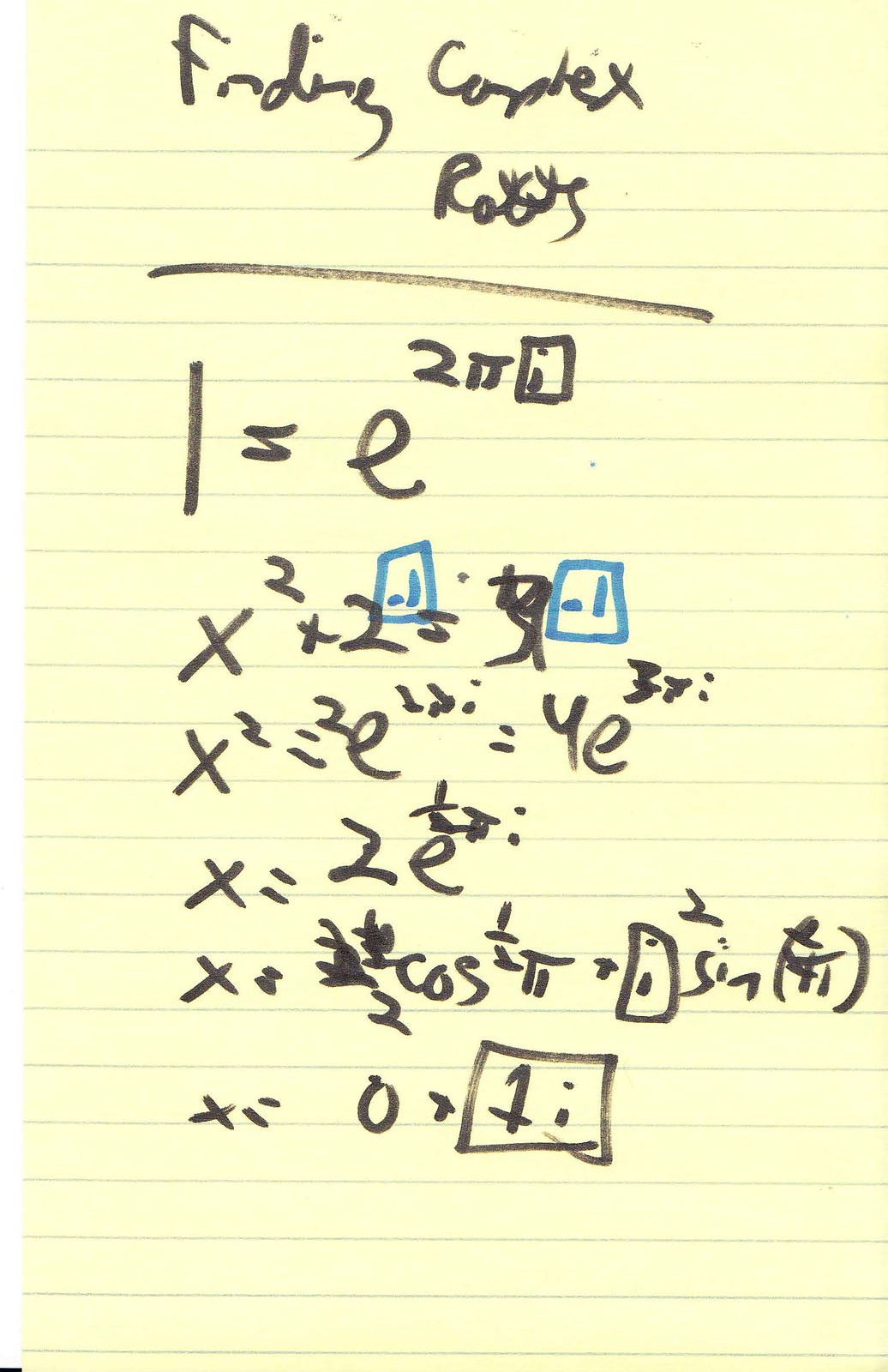This image captures a yellow lined sheet of paper with black markings on it. At the top of the paper, written in cursive, is the phrase "Finding Complex Roots." Below this title, a horizontal line spans the width of the paper, clearly separating the title from the content underneath. The content consists of various mathematical problems written with a black marker, which makes it somewhat challenging to discern the details.

The first visible equation starts with "1 = e." Below it, another equation features "x² + 2 =", but the result is obscured due to being crossed out. The next line shows "x² = 2e," followed by an expression that translates to "equals ye." There are three more mathematical equations displayed underneath, each gradually becoming more complex and extending off the visible part of the paper, making them harder to decipher. Overall, this sheet appears to be focused on solving or discussing complex mathematical roots.